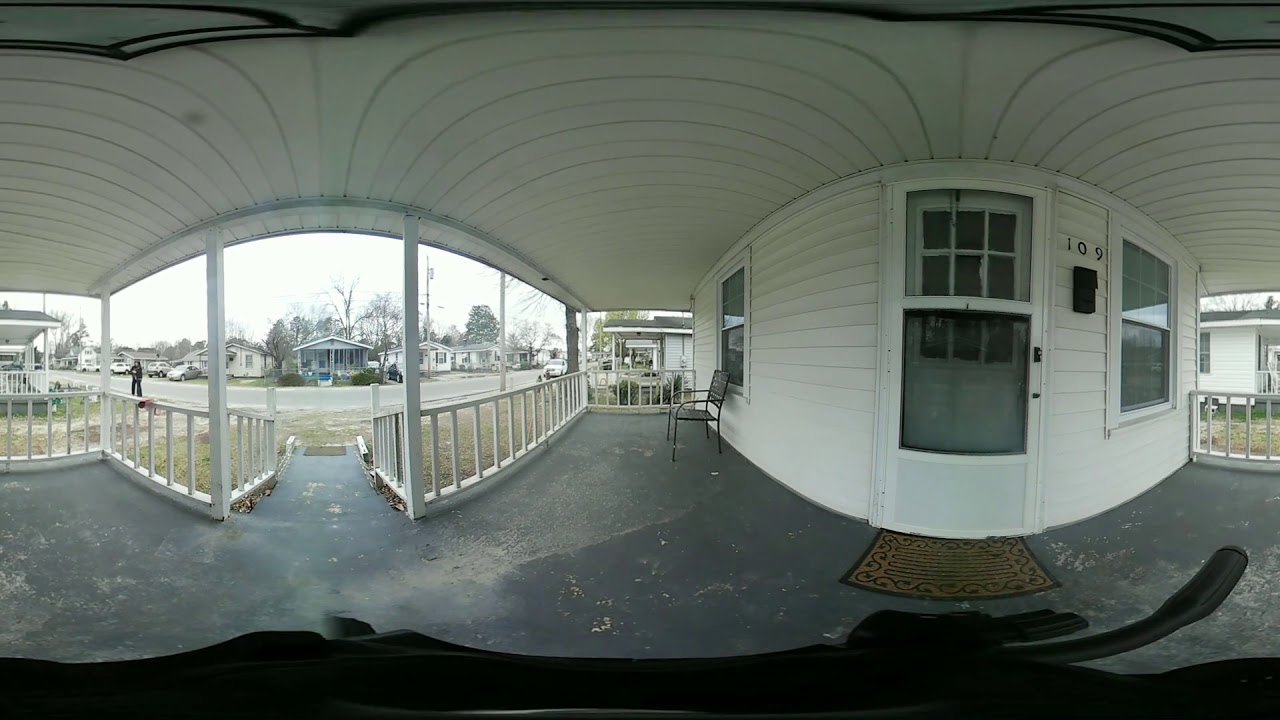The image is a wide-angle shot captured by a home security camera, depicting a front porch with a white ceiling streaked with light gray lines and a concrete floor that appears black and dirty. Central to the image, there's a white screen door with open panels at the top and bottom, covered by a mesh screen. The screen door leads to a white door with nine glass panes. To the right of the door, the number 109 is prominently displayed above a small black mailbox. Adjacent to the mailbox is a closed window with a white frame and two panes.

The porch has white railings, with white boards and poles supporting them. A throw mat lies directly in front of the door, and a ramp extends from the porch downwards. On the street beyond the porch, there's a person dressed in black clothing. The background also includes a view of neighboring houses with arched roofs, some trees, and visible power lines. Outside the porch area, elements such as a stone surface, a chair, some grass, and additional homes are discernible. The scene is set in daylight, framed as if someone is standing on their front porch.